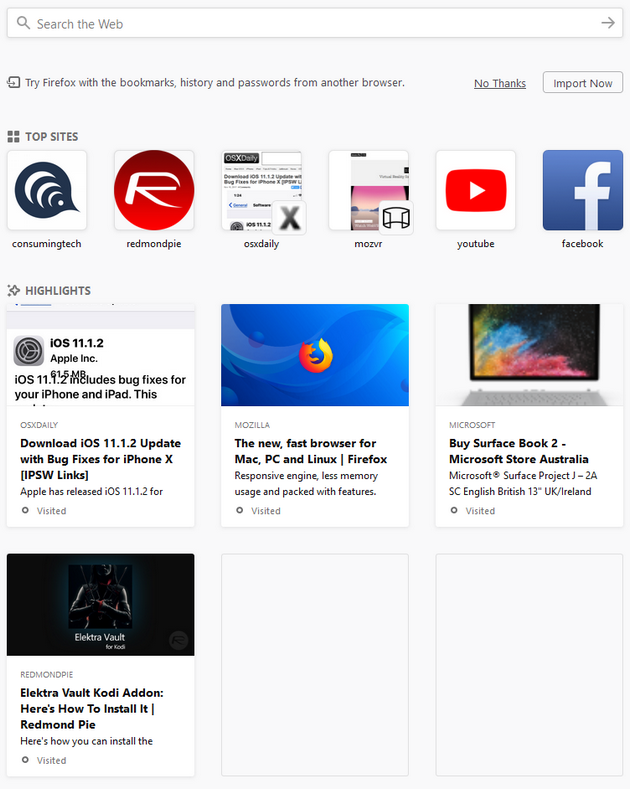In the image, the top section features a search bar labeled "Search the web" set against a light grey background. Below this search bar, there is a prompt encouraging users to "Try Firefox" by importing bookmarks, history, and passwords from other browsers. This prompt is followed by two options: an underlined "No thanks" and a button labeled "Import now."

Further down, the page is divided into sections. The first section is titled "Top Sites" and contains six squares, each holding an icon. From left to right, the icons represent the following sites: Consuming Tech, Redmond Pie, OSX Daily, Moz VR, YouTube, and Facebook.

Beneath the "Top Sites" section is another section titled "Highlights," which includes a box detailing information about the iOS 11.1.2 update from Apple Inc. This description reads, "iOS 11.1.2 includes bug fixes for your iPhone and iPad." Following this, there is additional text promoting the download of the iOS 11.1.2 update, mentioning that it includes bug fixes for the iPhone X and providing IPSW links for the releases.